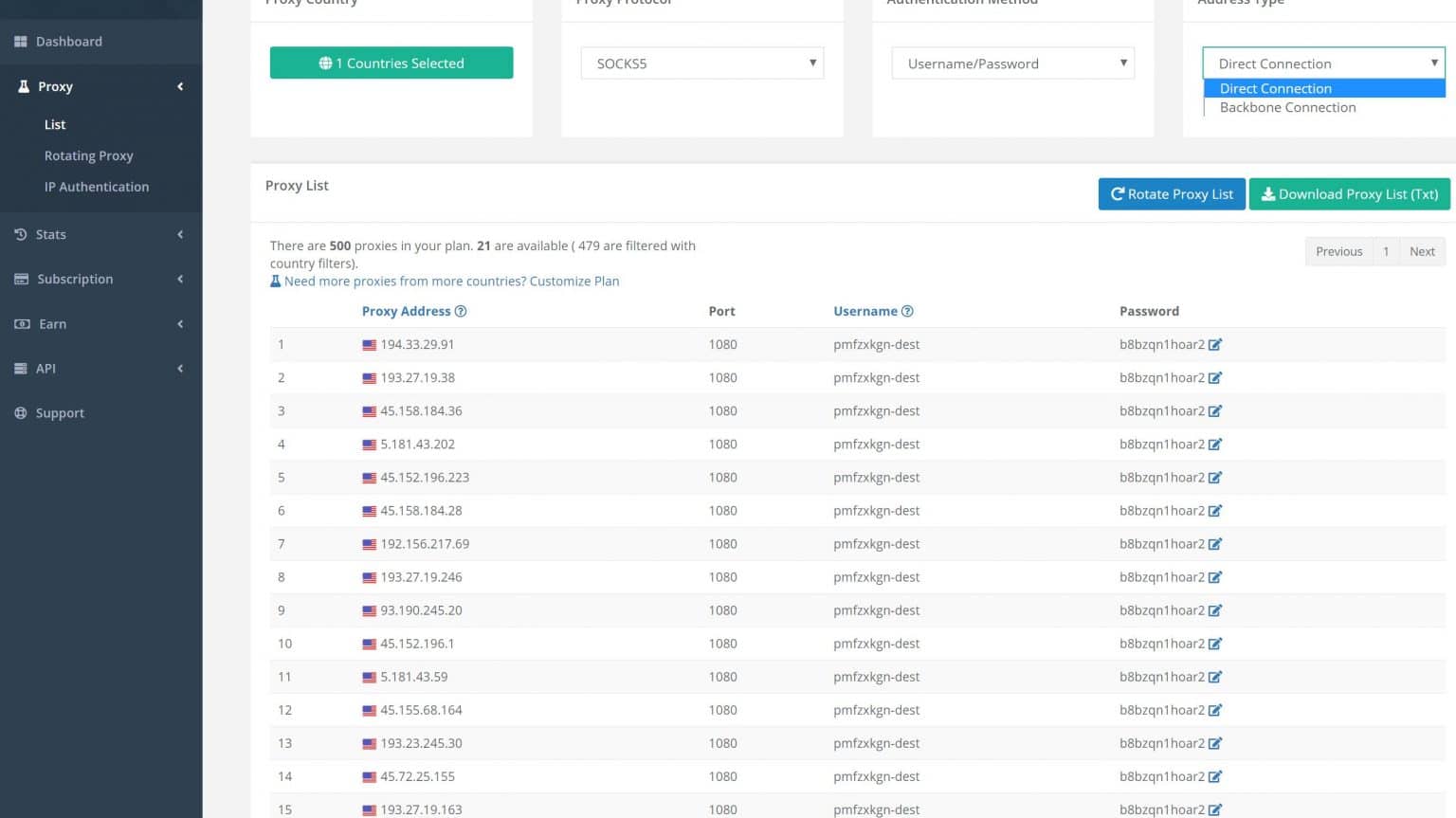This image depicts a section of a VPN interface focused on proxy server settings specifically for U.S. addresses. The screen features a comprehensive list under the heading "Proxy List," detailing ports, usernames, and passwords for various U.S.-based proxy servers. On the dashboard, there are options for "Restoring Proxy IP Authentication" and reviewing "Stats" related to VPN usage. Additionally, there's a section for managing subscriptions. Although the text detailing individual proxies is small and somewhat blurred, it is evident that there are 21 proxies listed, with 15 visible on the current display. This setup allows users to switch between available proxies, enhancing their online privacy and security by masking their internet activities.